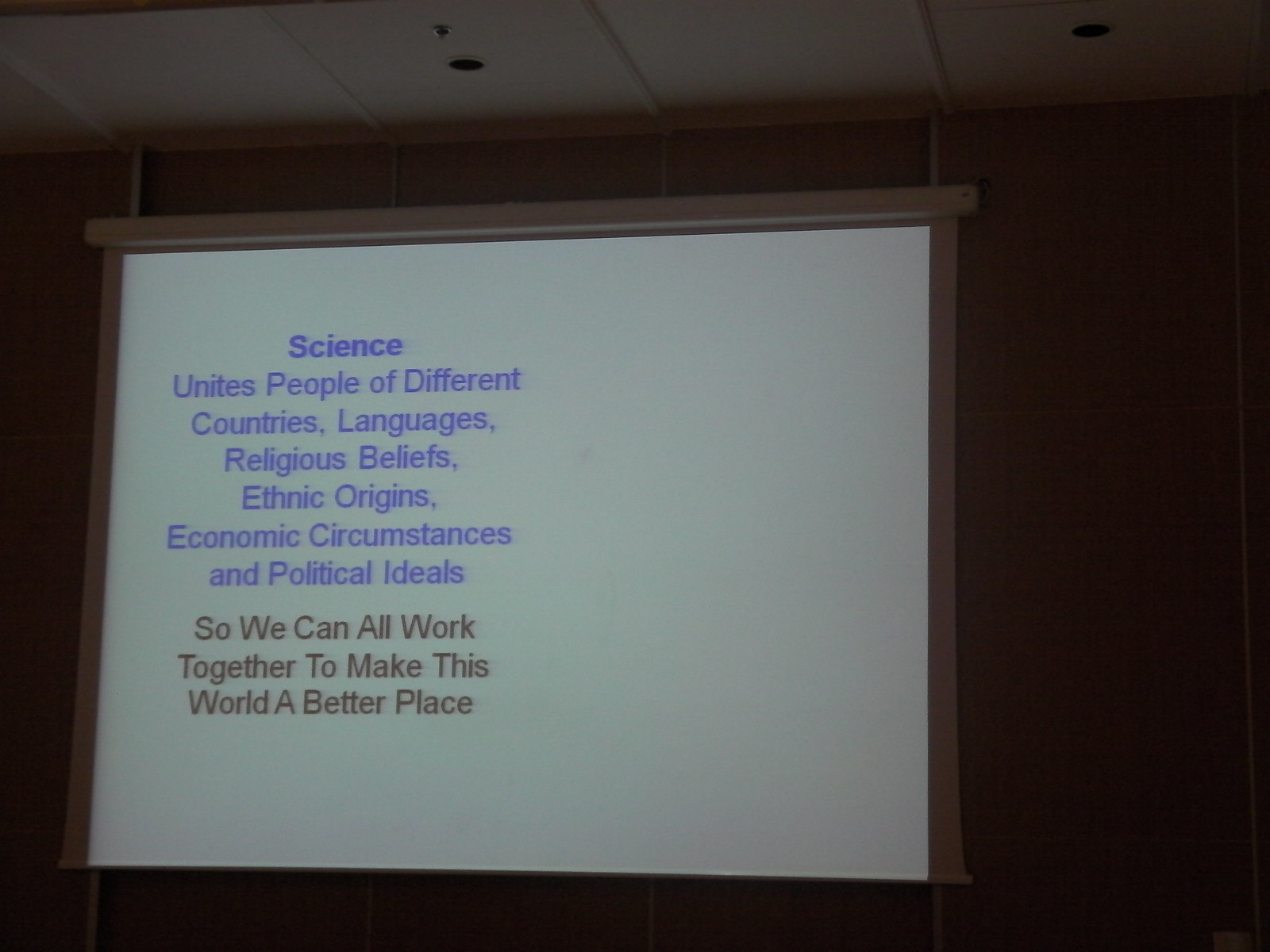In the dimly lit interior of a building, a photograph captures a projector screen suspended from the ceiling. The screen is centrally illuminated, displaying a slide with a white background adorned with text. The message, written in light purple at the top and black at the bottom, reads: "Science unites people of different countries, languages, religious beliefs, ethnic origins, economic circumstances, and political ideals. So we can all work together to make this world a better place." Surrounding the brightly lit screen, the dark room and suspended ceiling frames the image, emphasizing the importance of the projected words.